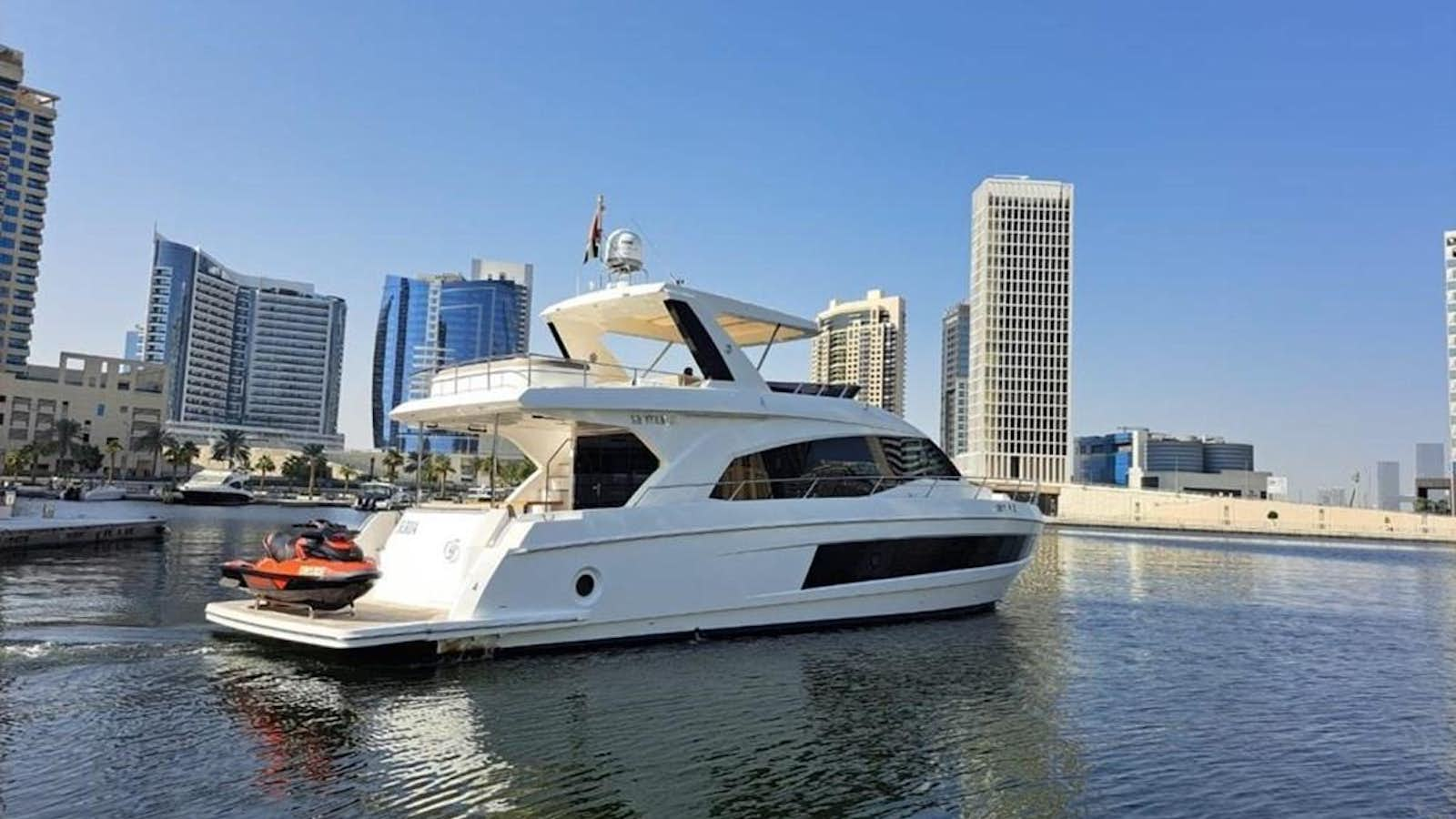This vibrant image captures a sleek white yacht cruising to the right. On the yacht’s back deck sits a red jet ski, and the vessel features tinted windows, an upper deck with a roof for shade, and some communications equipment on top. The setting appears to be a calm, vast body of water—possibly a lake or ocean—reflecting the clear, blue, cloudless sky. Along the edge of the water, palm trees add a tropical touch, and in the background, a skyline of tall buildings and skyscrapers hint at a distant downtown area. The serene scene is devoid of people or cars, with only a small boat faintly visible near the shore.